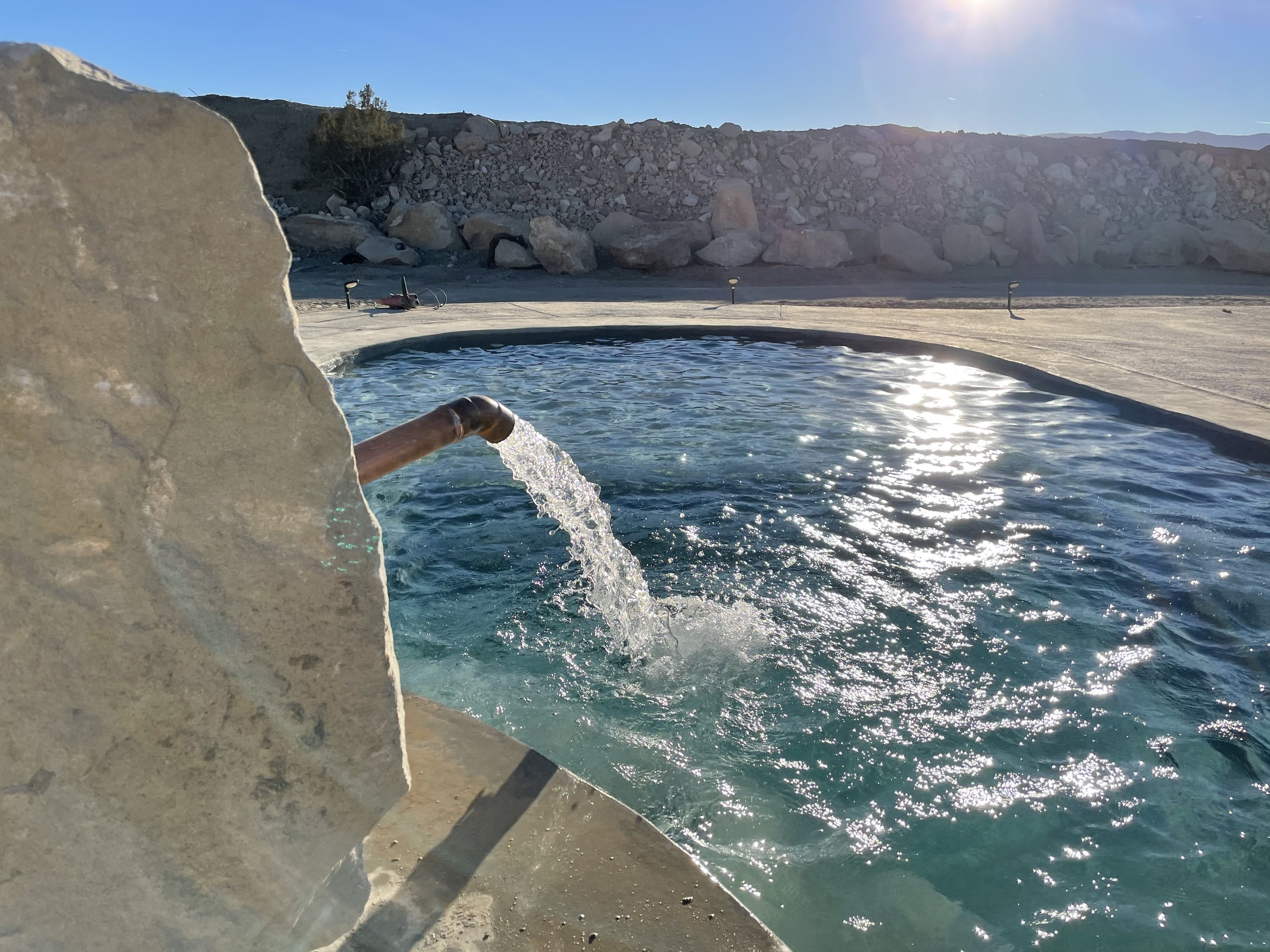This vertical rectangular photograph captures a serene outdoor reservoir scene on a sunny day, characterized by its natural light and clear blue sky occupying the upper portion of the image. Central to the composition is a well-defined, oval-shaped concrete pool filled with pristine, clear water, so transparent that the bottom is visible and even a step can be discerned. A prominent feature is a large pipe extending from a stone or concrete structure—resembling a massive boulder—on the left side, from which water cascades gracefully into the reservoir. The pipe casts a noticeable shadow on the surrounding dry, cemented area, enhancing the sense of bright daylight. The background comprises a pile of rocks and boulders, with larger ones at the base supporting smaller stones atop them, giving a rugged texture to the scene. This dry, sunlit setting contrasts sharply with the inviting clarity of the water, making the pool appear especially refreshing. Just a hint of the sun can be seen in the upper right corner, further emphasizing the bright and arid environment.